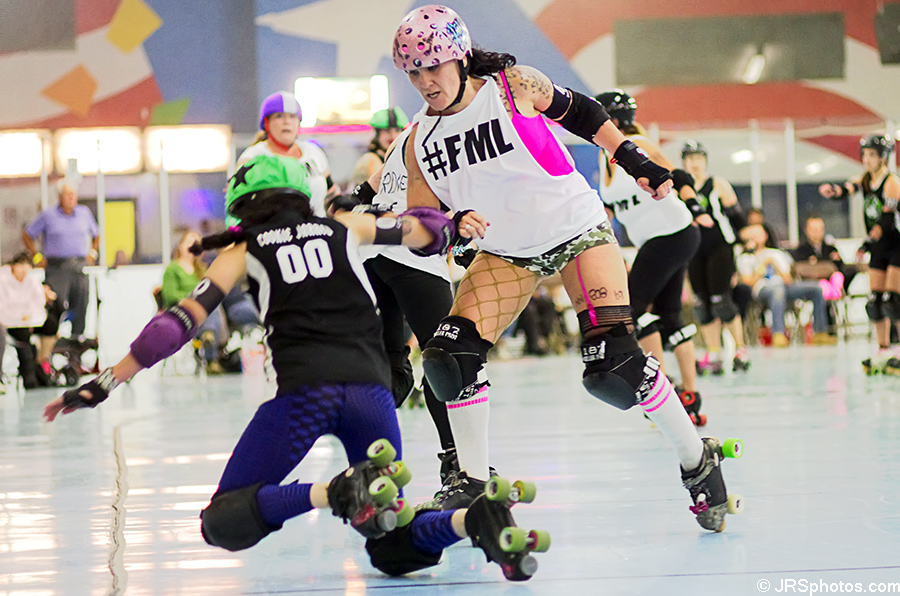This vibrant color photograph captures an intense moment in a roller derby match, showcasing two female skaters from opposing teams in mid-action. The skater in the foreground, marked by her black jersey bearing the number 00, is on her knee, seemingly having been knocked down. She is outfitted with protective gear, including knee and elbow pads, and a green helmet adorned with a single black star. Her tights and dark skates add to her team's uniform. Opposite her, an offensive player from the other team stands tall, appearing to initiate the confrontation. This skater dons a white sleeveless t-shirt emblazoned with the hashtag FML, paired with a distinctive pink helmet and black armbands. Both athletes are surrounded by the bright and bustling atmosphere of a roller rink, its white floor standing out under vibrant lights. In the background, other skaters and spectators on benches add to the lively and competitive ambiance of this women's roller derby event.